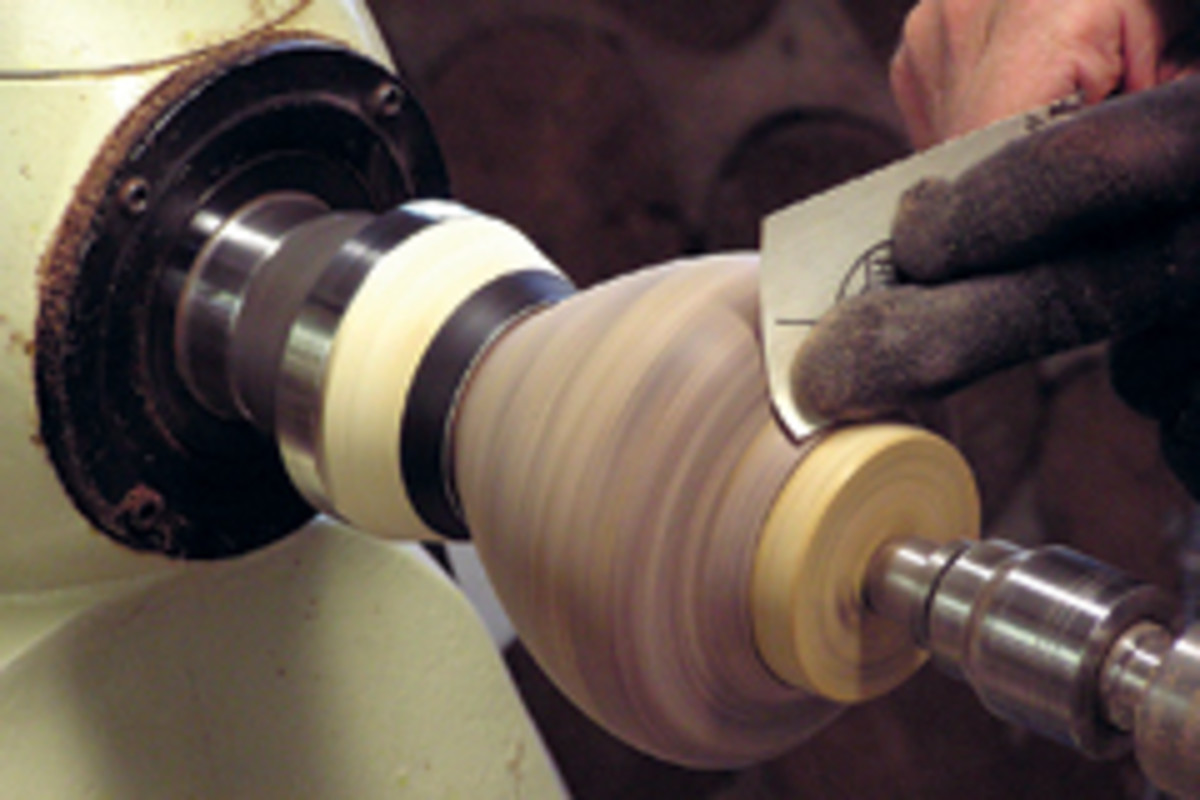In this close-up image, a woodworking lathe is holding a beautifully grained urn-like wooden object, which appears to be in the process of being sanded down. The wood showcases a tan, sand-washed hue with intricate grain patterns. A person is meticulously polishing the wood using a piece of sandpaper, with their left hand clad in a black glove and their right hand bare. Their left hand holds the back of the sandpaper while the right hand holds the opposite end further from the spinning lathe. The lathe features metallic parts at each end, contributing to its polished, industrial look, and the piece of wood is securely held between these components. The image exudes a sense of craftsmanship and precision, highlighting the detailed process of woodworking within what is likely a workshop setting.